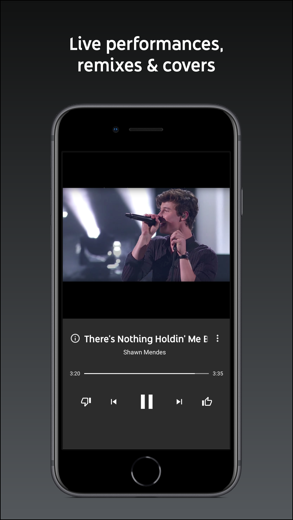A detailed photograph captures a slightly older cell phone resting on a gradient background that transitions from medium gray at the bottom to dark gray, almost black, at the top. Overlaid on the background, in the top quadrant, is bold white text reading "Live Performances, Remixes, and Covers."

Beneath this text, the cell phone with a steely gray bezel is displayed prominently. The phone features a black portion at the top and bottom, including a round button at the bottom and a gray, pill-shaped speaker at the top. Positioned to the left of the speaker is the front camera, encased in a bluish-tinged circle.

On the screen of the phone, a combination of elements is superimposed. The upper half of the screen displays a photograph of a man with short, curly brown hair, wearing a shirt with rolled-up sleeves, holding a microphone to his mouth. Bright spotlights illuminate the background behind him. 

Directly below the photograph is a gray section with text. At the top of this section, partially cut off, are the words "There's Nothing Holding Me," followed by the name "Shawn Mendes". At the bottom, a music progress bar is visible, showing 3 minutes and 20 seconds elapsed on the left and a total duration of 3 minutes and 35 seconds on the right. The progress bar is filled with white to indicate the portion of the song that has been played.